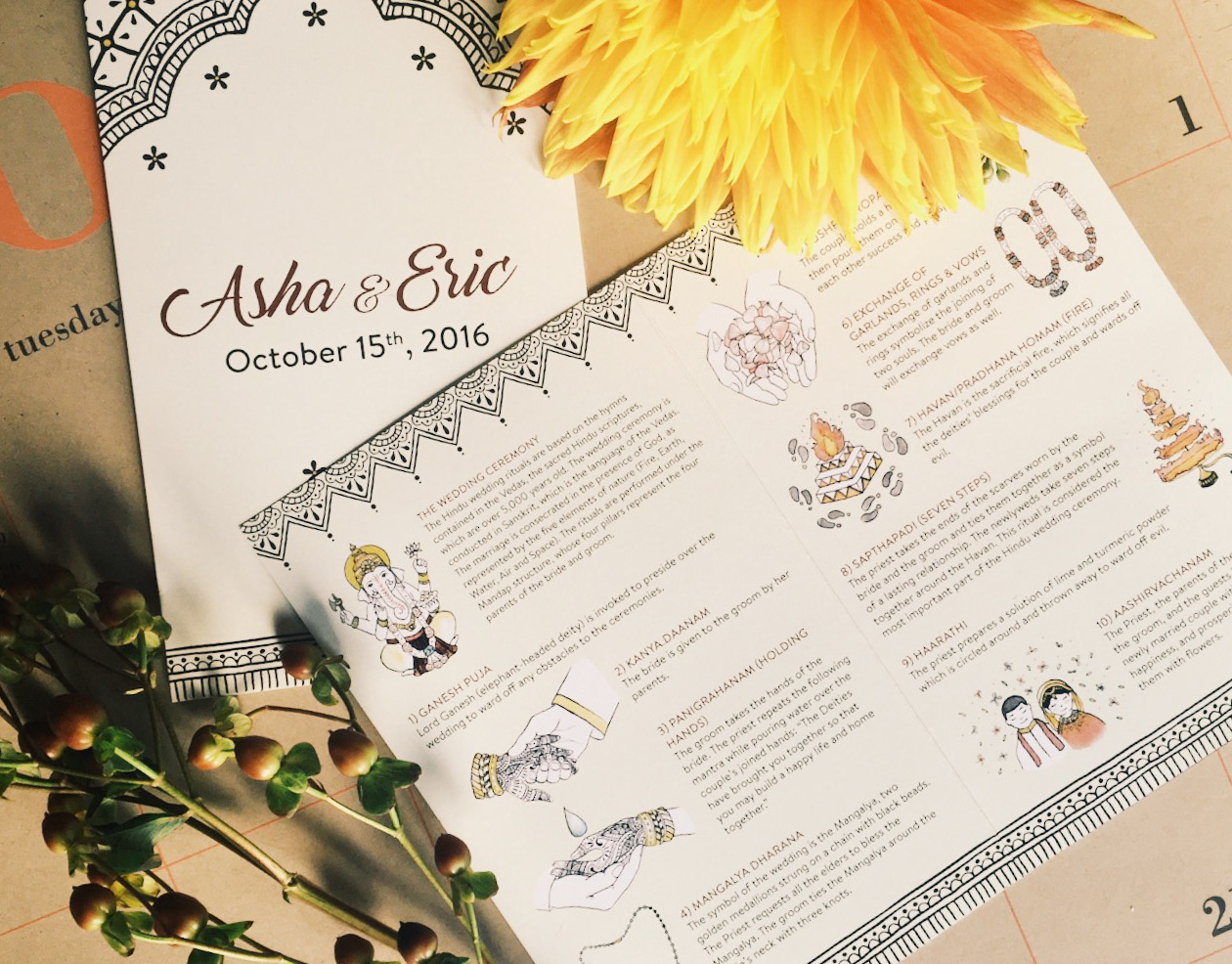The image captures a top-down view of a wedding invitation and an informational pamphlet laid out on a tan-colored desktop calendar. The focal point is a closed white pamphlet adorned with a black scalloped and star border. It features the text "Asha and Eric, October 15, 2016" in dark red and black lettering. The pamphlet is placed alongside an open piece of paper showing detailed illustrations and paragraphs, depicting elements of a traditional Hindu wedding, including images of the Hindu god Ganesh, hands with henna tattoos, and wedding jewelry. The calendar beneath shows part of the word "Tuesday" and the number "1" in black text on the left edge. Decorative elements in the image include a half-visible large yellow flower in the top center, and green sprigs with small brownish buds and flowers that have not yet bloomed in the lower left corner.